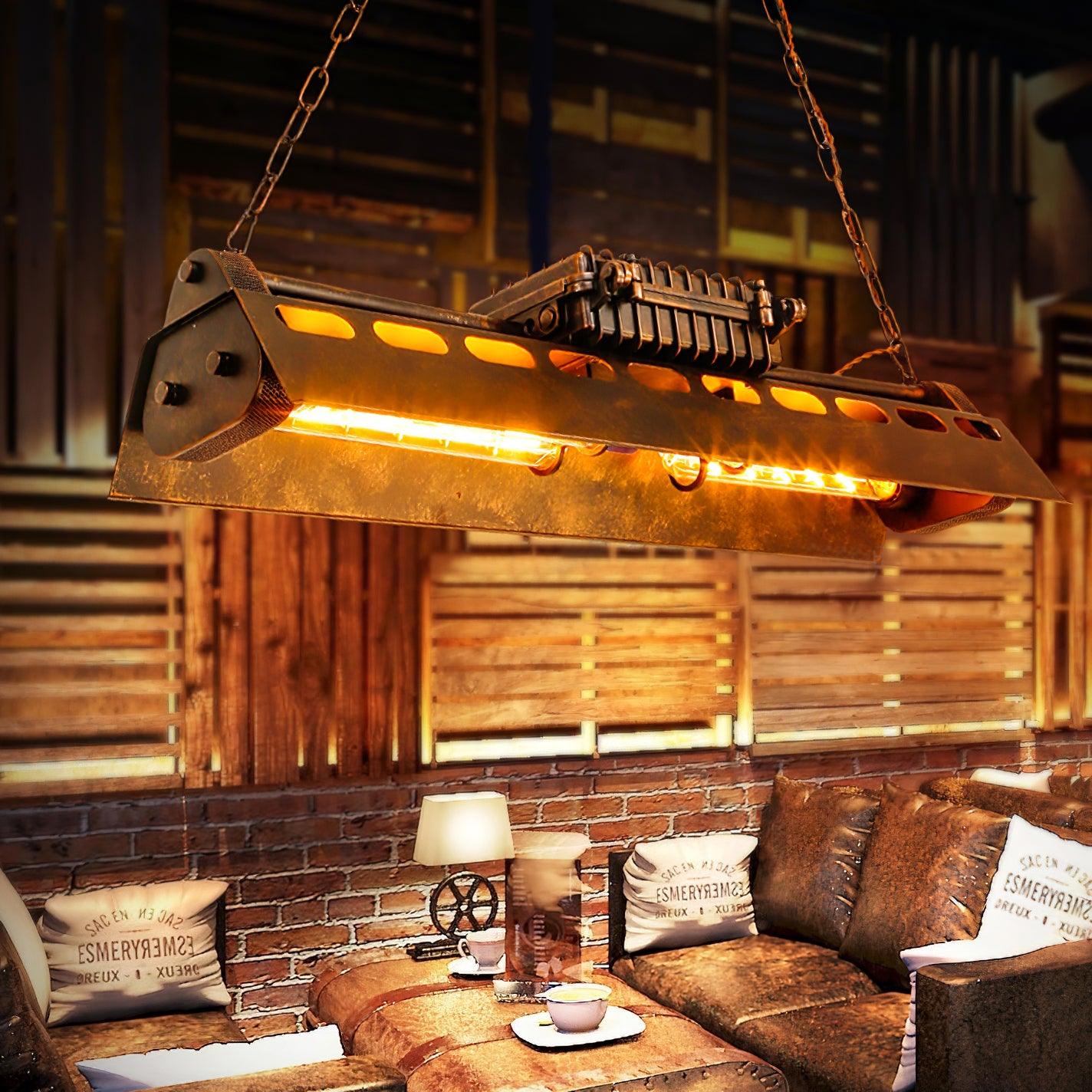The photograph depicts an industrial-themed, boutique coffee shop with a distinctive steampunk vibe. The seating area features two distressed brown leather couches, facing each other, equipped with throw pillows that display the letters "E-S-M-E-R-Y" arranged in various directions. Between the couches sits a makeshift table, crafted from what appears to be an old treasure chest or steamer trunk, complete with brown leather straps. On the table, there are two coffee cups on plates, a small rustic lamp fashioned from metal gears, and a menu angled between the cups.

The decor is highlighted by red brick walls with prominent grey grouting and wooden slats or pallets arranged at varying orientations, providing a rugged backdrop. A unique industrial lamp, resembling a modified heat lamp with an almost steampunk design, hangs from the ceiling, suspended by rusted chains. The lamp features a brass and rusted metal body with fluorescent lights giving off a yellowish-orange glow, enhancing the ambient lighting in the space. Overall, the area combines vintage elements with a hipster, bohemian atmosphere, making it a cozy and trendy spot for coffee patrons.